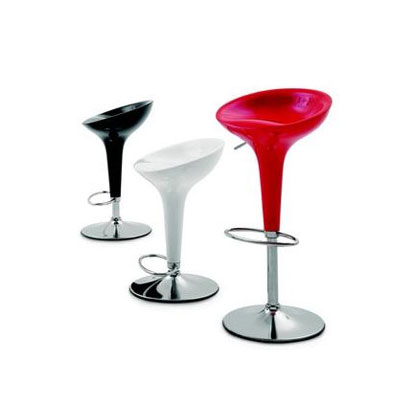The photograph showcases three modern, adjustable stools aligned against a white background. Each stool features a sleek, curved seat without a backrest, designed for simplicity and comfort. All stools are equipped with chrome stands and bases, as well as circular footrests. The stools vary in height, indicating their adjustable nature. The stool on the left is black, the one in the middle is white, and the one on the right boasts a red or deep pink seat. The minimalist design emphasizes their functionality and aesthetic appeal, with the chrome elements adding a touch of modern elegance.